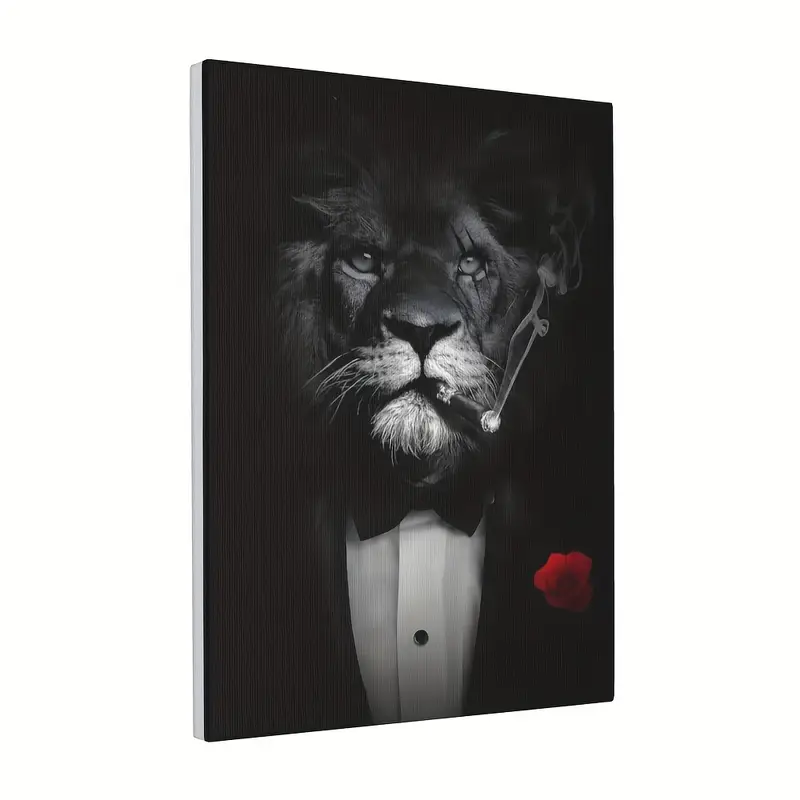In this striking portrait reminiscent of a scene from "The Godfather," a lion is depicted with a distinctively sophisticated and yet gritty demeanor. Dressed in a meticulously detailed black and white tuxedo, complete with a black bow tie and a red rose adorning his coat pocket, this lion exudes an air of elegance and power. He has a cigar clamped between his teeth, with smoke curling up around his chiseled face, enhancing his fierce yet refined look. The lion’s chin and upper lip are white, accentuating his prominent whiskers while his slightly disheveled mane reveals his small, cubby cat ears. Notably, there are deep scars slashing across his left eye, suggesting a past filled with battles and resilience. This artwork, performed on a canvas and set against a simple white background, is slightly tilted, adding an additional layer of intrigue and defiance to the overall composition. The portrait captures the lion from the chest up, framing his intense gaze directly at the viewer, embodying a timeless and commanding presence.